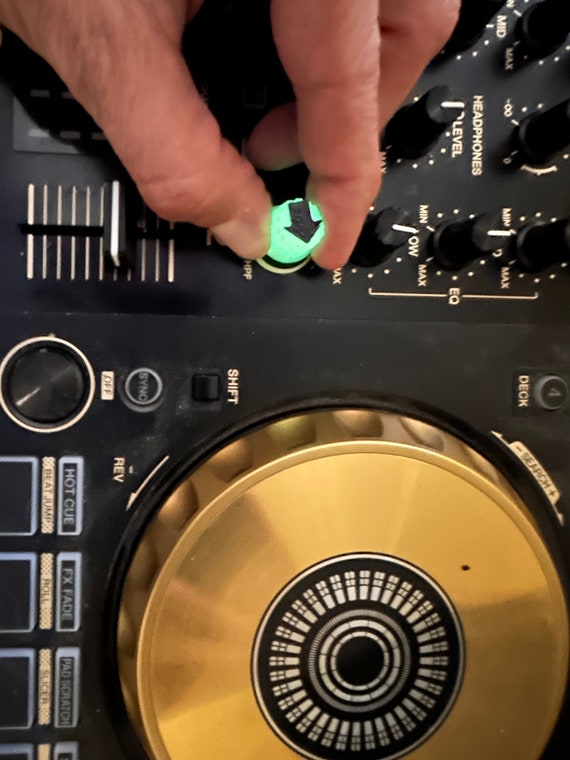The image presents a detailed, overhead view of a DJ mix table, primarily black in color, with a myriad of dials and buttons. Central to the scene is a man's hand, likely his index finger and thumb, skillfully adjusting a neon green, illuminated knob marked with a black arrow. Around this knob, various labels such as "min," "max," and "headphone levels" can be seen in white text against the black background. The table features a large golden disc, possibly a record player, positioned at the bottom half of the photo, adorned with a black circle and white markers at its center. Additional controls and buttons labeled "hot cue," "FX fade," "pad," "sync," "shift," "deck," and "scratch" are scattered throughout the board, catering to nuanced sound modulation. The image is vibrantly colored, with prominent shades of black, gold, and green, and is brightly lit, offering a clear and organized portrayal of the DJ equipment.